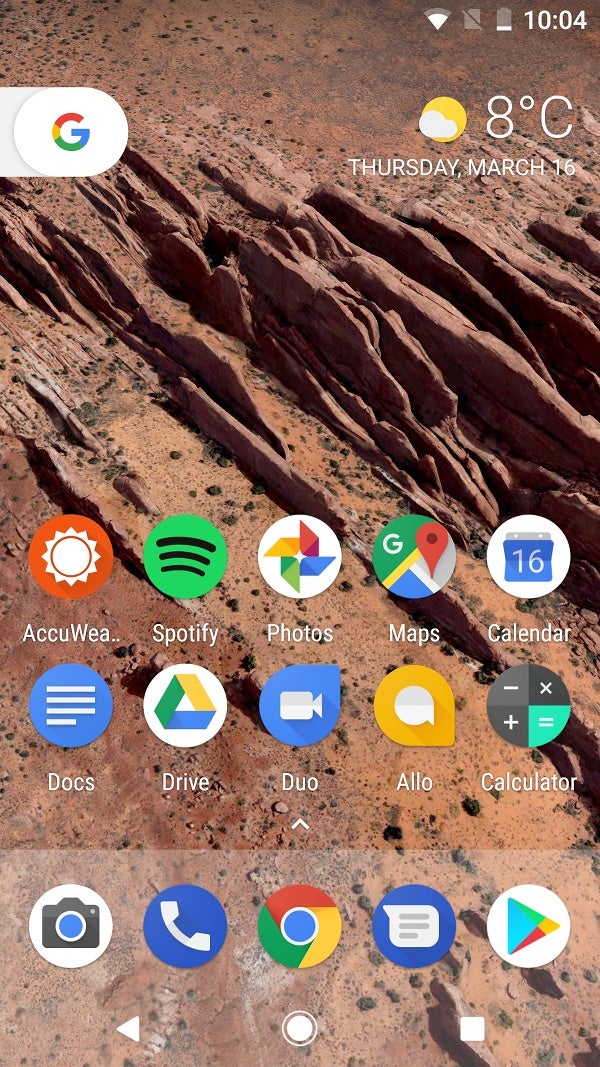Captured on a cell phone, this image depicts a rustic, desert-like landscape characterized by thin, brown rock formations jutting upward, resembling shale. The screen displays a temperature of 8 degrees Celsius and the date as Thursday, March 16th. Notably, the battery indicator at the top shows a critically low level with only a sliver of white remaining. The current time, visible in the upper right-hand corner, is 10:04 AM.

On the left side of the screen, a multicolored "G" icon representing Google is prominent. Below that, three rows of app icons are neatly arranged, each accompanied by its name. The first row includes AccuWeather, Spotify, Photos, Maps, and Calendar. The second row features Docs, Drive, Duo, Allo, and Calculator. The bottom row contains quick-access icons for the Camera, Phone application, Google Chrome, a speech box (possibly for messaging or voice commands), and Google Play. This detailed layout offers a snapshot of the user's home screen amidst a striking natural backdrop.